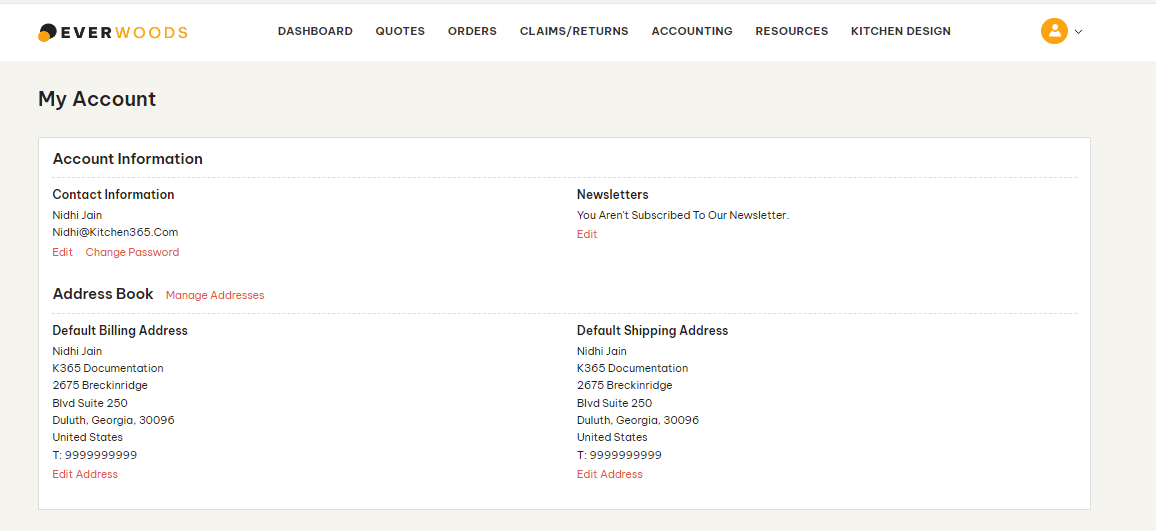The screenshot features a user dashboard for Ever Woods, prominently displaying the brand name at the top in all-capital letters, with "EVER" in black and "WOODS" in orange. Below the header, there are navigation options including: Dashboard, Quotes, Orders, Claims/Returns, Accounting, Resources, and Kitchen Design. 

The account section provides detailed account information for Nidhi Jain, spelled N-I-D-H-I J-A-I-N. It lists the email address as nidhi@kitchen365.com, with options to edit the information or change the password. The newsletter section indicates that the user is not subscribed to any newsletters, with an option to edit this setting.

The address book portion shows both the default billing and shipping addresses as follows:

**Default Billing Address:**
- Name: Nidhi Jain
- Company: K365 Documentation
- Address: 2675 Breckenridge Boulevard, Suite 250, Duluth, GA 396, United States
- Telephone: 999-999-9999
- Option: Edit Address

**Default Shipping Address:**
- Name: Nidhi Jain
- Company: K365 Documentation
- Address: 2675 Breckenridge Boulevard, Suite 250, Duluth, GA 396, United States
- Telephone: 999-999-9999
- Option: Edit Address